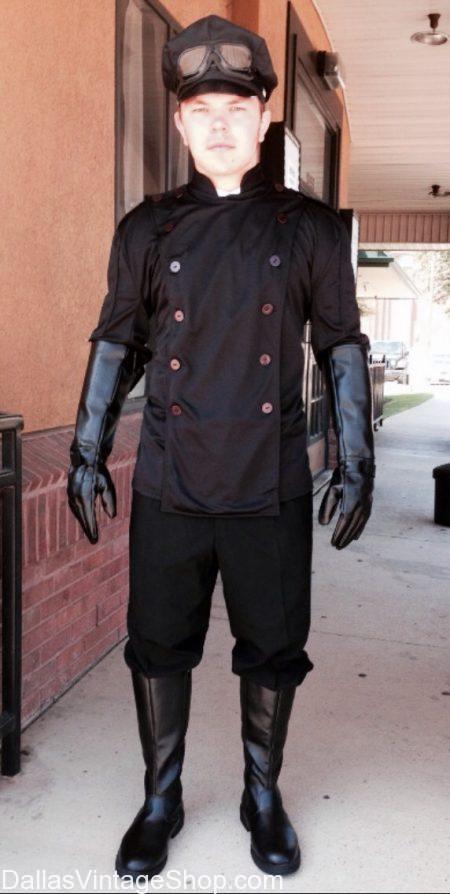The image portrays a serious-looking, pale-skinned man dressed in a head-to-toe black outfit, comprising a double-breasted button-down shirt, long pants tucked into knee-high boots, and elbow-length gloves. He also sports a raised black hat with aviator-style goggles perched on top. He has red eyebrows and hair, adding a touch of color against his predominantly black attire. The man stands on a concrete sidewalk in front of a building featuring a mix of dark tan stucco, red bricks at the base, and a white wooden ceiling with silver recessed lights, suggesting a front porch area. The background is bathed in sunlight, highlighting both the building's terracotta elements and the man's distinct features. The photo includes the text "DallasVintageShop.com" in white at the bottom, hinting that this image may be associated with a vintage or costume shop.